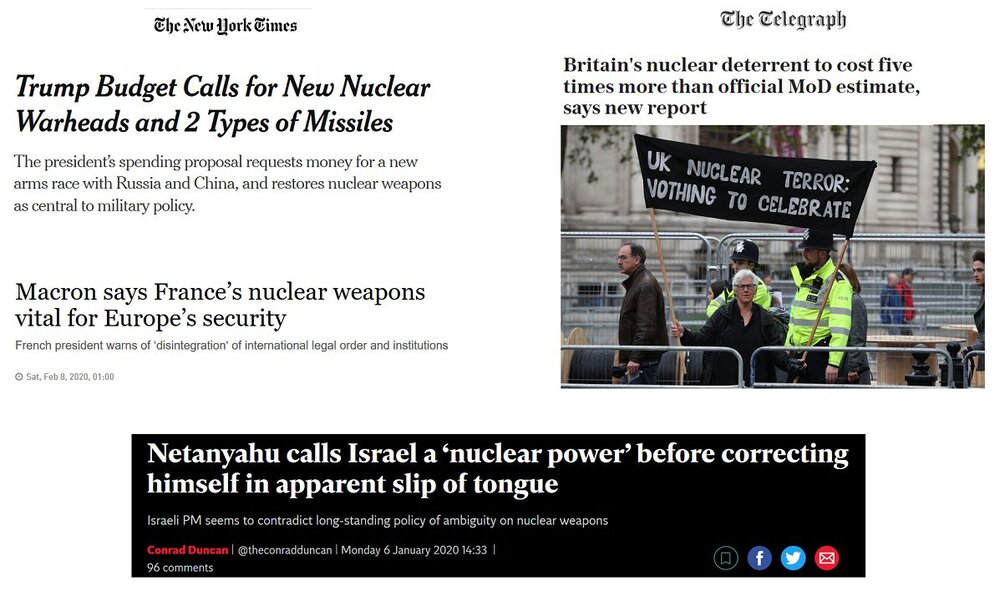A collage of various news headlines on a white background, interspersed with related imagery, captures modern concerns on nuclear armaments and political discourse:

1. **Top Left Corner**: A New York Times article titled *"Trump Budget Calls for New Nuclear Warheads and Two Types of Missiles"* details the president's request for an increased budget to fuel a new arms race with Russia and China. The subtitle reads, *"The President's Spending Proposal Requests Money for a New Arms Race with Russia and China and Restores Nuclear Weapons as Central to Military Policy."* The New York Times logo and title are prominently displayed in bold, while the subtitle is in regular black text.

2. **Top Right**: The Telegraph's headline asserts, *"Britain's Nuclear Deterrent to Cost Five Times More than Official MOD Estimate, Says New Report."* Below the headline is an evocative image of a peaceful protester holding a black banner with silver text proclaiming, "UK Nuclear Terror Voting to Celebrate."

3. **Bottom Left**: Another screen grab highlights a controversial statement by Israeli Prime Minister Netanyahu. The headline reads, *"Netanyahu Calls Israel a Nuclear Power Before Correcting Himself in Apparent Slip of Tongue,"* with the subtitle, *"Israeli PM Seems to Contradict Longstanding Policy of Ambiguity on Nuclear Weapons."* Accompanying social media sharing buttons for bookmarking, Facebook, Twitter, and email are visible at the bottom right of this image.

4. **Bottom Right**: An unspecified headline, lacking the source website’s identification, stands ambiguously above Netanyahu's headline, hinting at more layered discussions on nuclear strategies.

This collection underscores the ongoing international dialogues and controversies surrounding nuclear policies, captured through a series of compelling headlines and supporting visuals.